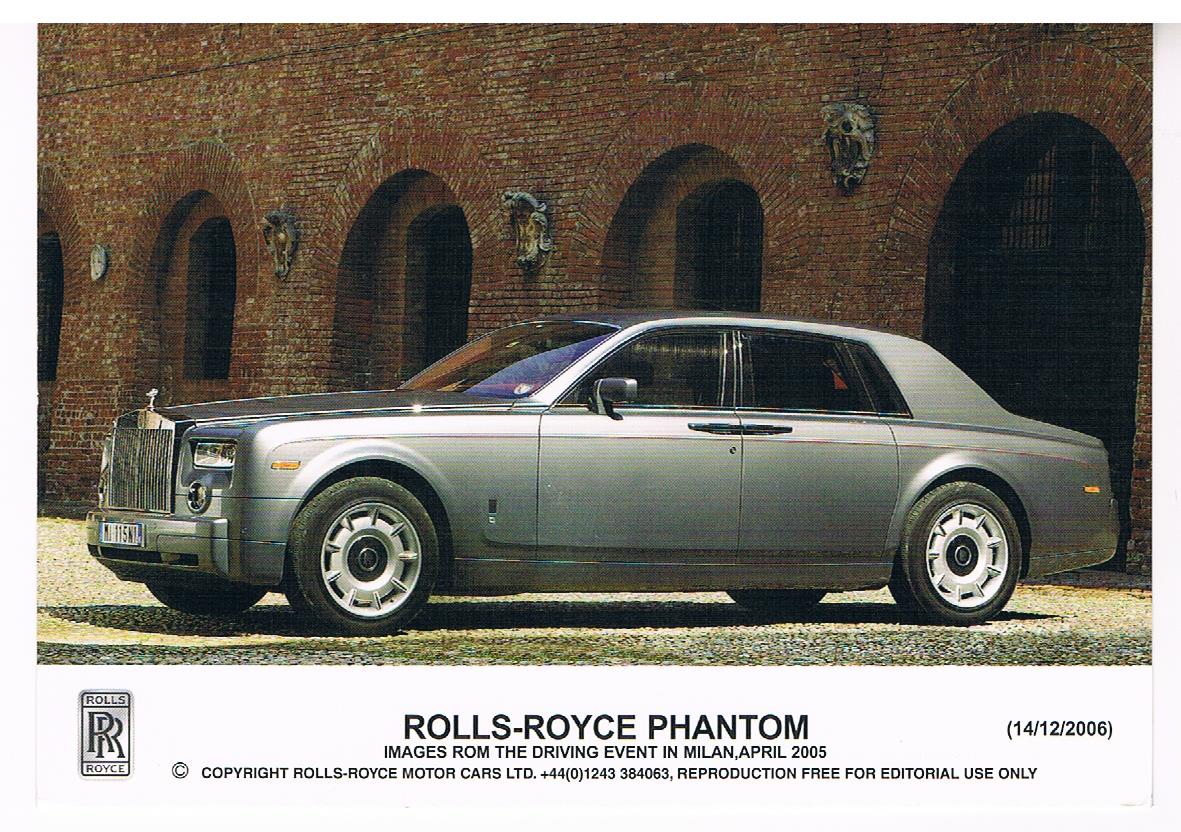The image depicts a side profile of a luxurious silver-gray 2005 Rolls-Royce Phantom parked in front of an ornate, large brick building with tall, arched windows and doorways, resembling a coliseum. The silver car, with its four doors and shiny, tall grille topped with the iconic hood ornament, is prominently featured. Text within the image, alongside the Rolls-Royce logo located at the bottom left, states "Rolls-Royce Phantom," and notes that these visuals are from a driving event held in Milan, April 2005. Below this information lies a copyright notice from Rolls-Royce Motor Cars Ltd. accompanied by a phone number, and a clause stating that the image is free for editorial use only. The setting is mid-day, with all the car windows rolled up, positioned gracefully on a stone-cobbled road.